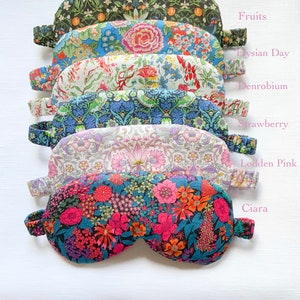This image showcases six brightly colored fabric sleep masks arranged in a vertical stack on a light blue background. Each mask features a unique and vibrant pattern, predominantly floral, with corresponding labels in pink text placed to the right of each mask. From top to bottom, the masks are named "Fruits," "Elysian Day," "Denrobium," "Strawberry," "Laudan Pink," and "Sierra." 

Starting at the top, the "Fruits" mask features a green background adorned with small orange motifs and white flowers. "Elysian Day" has a lighter blue background, dotted with both large and small floral prints in pink, red, and green hues. The "Denrobium" mask displays a white backdrop with various mixed-colored splotches in green, red, and blue. 

Next is "Strawberry," which comes with a blue background and white floral designs. Below it, "Laudan Pink" presents a lilac background embellished with pink flowers. The bottom mask, "Sierra," boasts a bright blue backdrop with pink and orange flowers, along with smaller pink and green floral accents. 

The sleep masks are seamlessly stacked, showcasing their vivid patterns and colors, making them visually appealing and neatly organized.